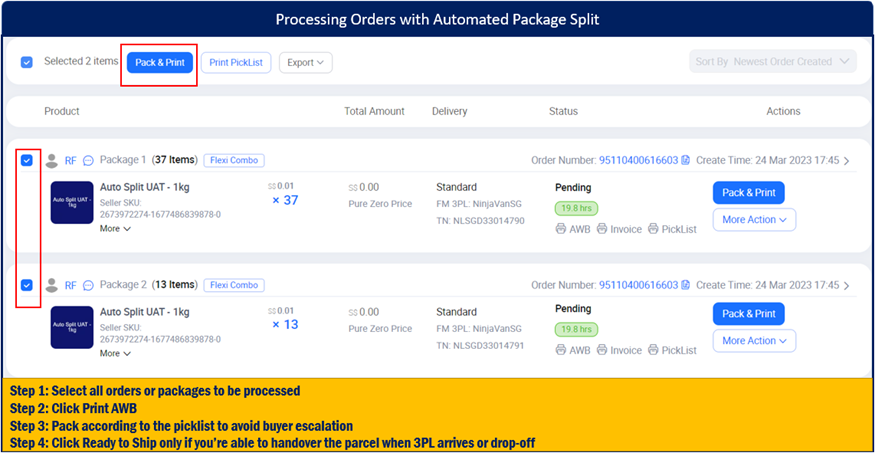This is a detailed caption for the provided image:

---

The image is a screenshot of a website interface designed for processing orders with an automated package split feature. The visual design prominently features white and dark blue colors. A dark blue header spans across the top of the page, encapsulated by a thin dark blue border surrounding the entire page. Just below this header, the page instructs users to "Select two items."

Highlighted in a bright blue color, with a red outline, is the "Pack and print" button, drawing immediate attention. To its right, there is a "Print pack list" option followed by an "Export" drop-down menu, indicating functionality for exporting data.

The main content area displays information about two pending orders, both of which have been checked off, suggesting they are selected for processing. On the far left, small checkboxes correspond to each item. The details for the orders include:

- Package one: 37 items, designated as a "Flex combo" with "Auto split UAT-1kg."
- Seller SKU number underneath that.
- Additional attributes such as the amount, standard delivery method, order number, and the date and time the orders were created.

The bottom of the image features a prominent yellow box with dark blue text, outlining four essential steps for order processing:

1. Select all orders or packages to be processed.
2. Click "Print AWB" (Air Waybill).
3. Pack according to the pick list to avoid buyer escalation.
4. Click "Ready to ship" only if you are prepared to hand over the parcel when the third-party logistics (3PL) provider arrives or if you plan to drop it off.

This screenshot appears to be part of a tutorial page, providing users with a step-by-step guide on processing orders efficiently.

---